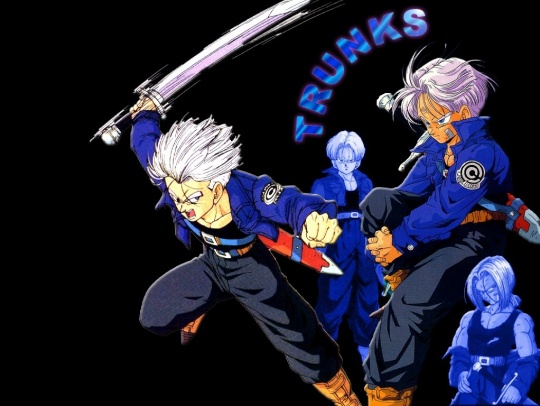This detailed caption merges all the shared and repeated elements from the voice descriptions into one cohesive, detailed narrative:

In the center of this animated drawing against a solid black background, the word "TRUNKS" is emphasized in bold blue letters with whitish-blue streaks, arranged in a semi-circle. The scene features four anime characters in a Japanese-style illustration, each sporting white hair. Dominating the foreground is a dynamic figure poised to strike with a futuristic sword, marked by a distinctive handle. He wears a blue jacket adorned with a "C" insignia patch on the left arm, black pants, a black tank top, and brown boots with buckles. A red sheath with a silver tip for his sword is slung across his back. To his immediate side is an almost identical character with slightly varied hair, dressed in the same attire. In the background, another character mirrors the first two in style, while the fourth figure displays longer hair. This final character’s jacket is draped loosely around their elbows, and they hold one knee against their chest with both hands. All four figures exude a determined, intense expression, contributing to the overall dramatic and hero-like atmosphere of the image.